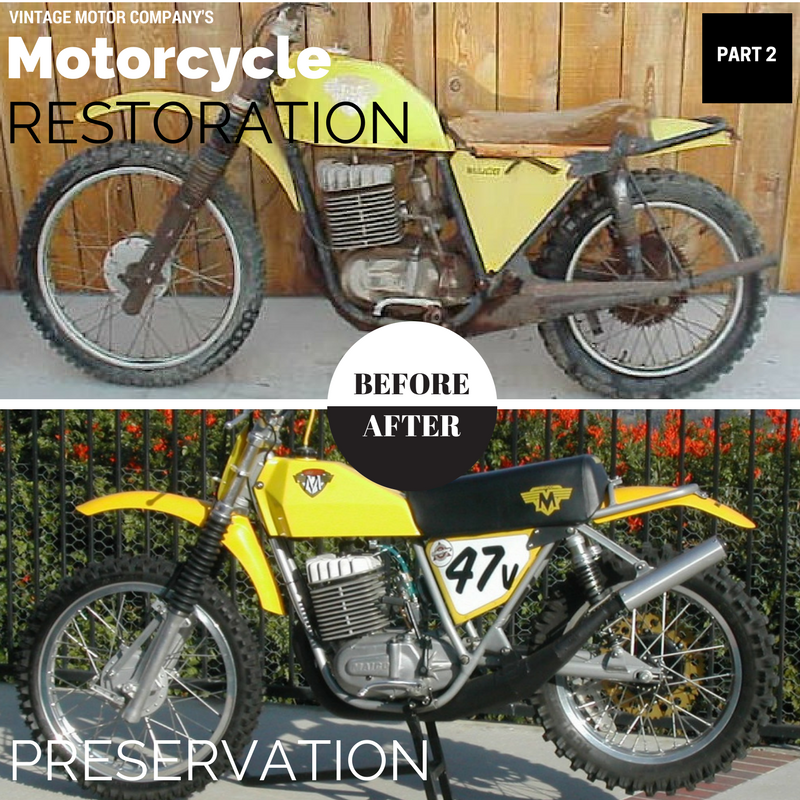The image is a before and after advertisement from Vintage Motor Company's motorcycle restoration series, indicated by text in the upper left corner. The upper section of the image depicts an old, run-down motorcycle with a yellow shell and exposed motor. The seat is worn and made of wood, and the wheels are dirty and worn. The metal parts appear rusty and the paint is faded. This scene is set against a bare wooden fence. 

In contrast, the lower section showcases the same motorcycle, now fully restored. The yellow color is vibrant, the motor is clean, and the tires are spotless. The restoration has returned the bike to a pristine condition, highlighted by the shiny and tidy appearance. The background here features a lush setting with flowers and vegetation, adding to the revitalized look of the motorcycle. Text in the upper right corner of this section marks it as 'Part Two' of the series. The central part of the image prominently features a circular graphic dividing the 'Before' and 'After' states, labeled accordingly, with 'Motorcycle Restoration' at the top and 'Preservation' at the bottom.